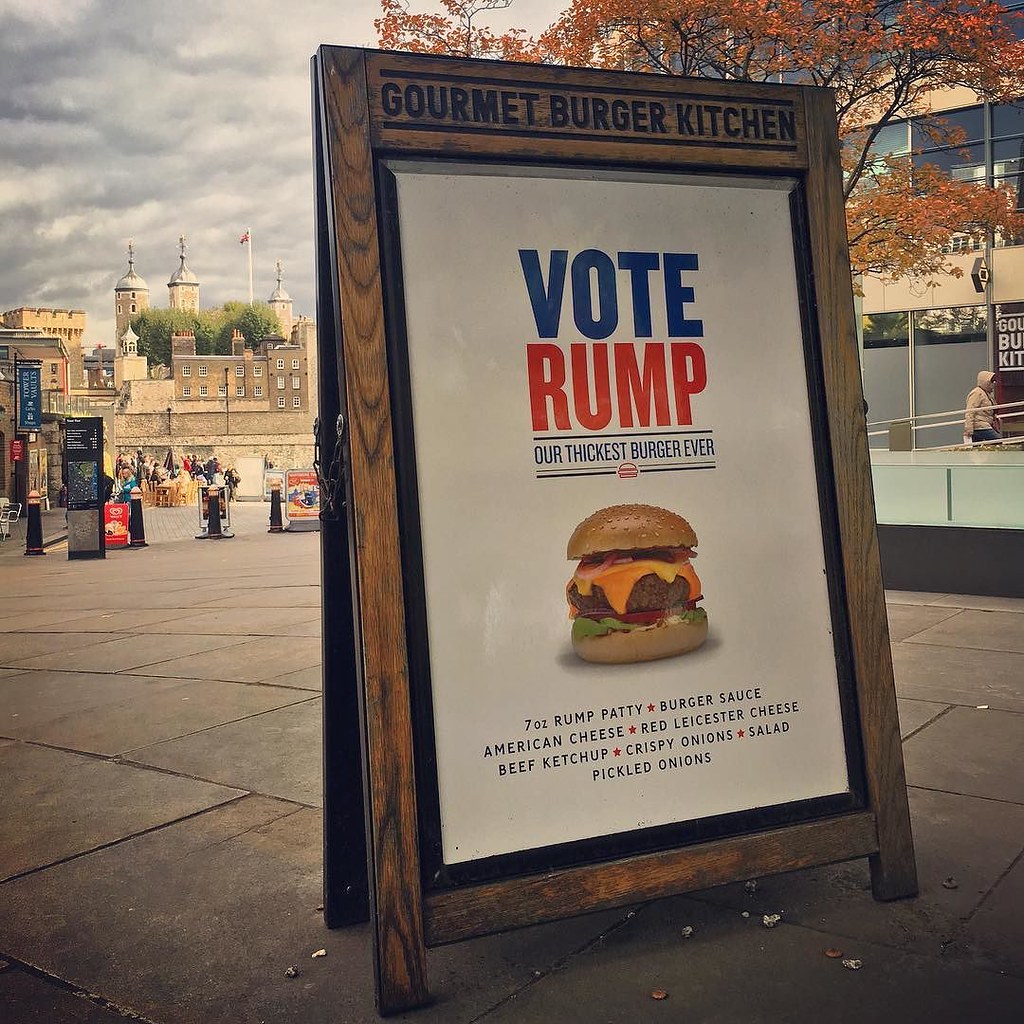The image features a wooden-framed standing poster board prominently placed on a tiled street. The sign, positioned to the right in the foreground, is topped with the words "Gourmet Burger Kitchen" etched in black on the wood. The central white poster is outlined in black and displays an advertisement in bold letters. At the top, "VOTE" is written in bright blue, followed by "RUMP" in red. Below it, a caption reads “Our Thickest Burger Yet.” An illustration of a large hamburger with a shiny sesame seed bun is showcased, featuring melted orange cheese, fresh lettuce, tomato, and possibly bacon. Underneath the image of the burger, text details the ingredients: "7-ounce Rump Patty," "Burger Sauce," "American Cheese," "Red Leicester Cheese," "Beef Ketchup," "Crispy Onions," "Salad," and "Pickled Onions," each separated by red stars. The background of the image, resembling a painting or drawing, depicts a cloudy grey sky above a street flanked by a large castle-like building on the left and modern structures on the right. Additional signs and people are seen in the distance.